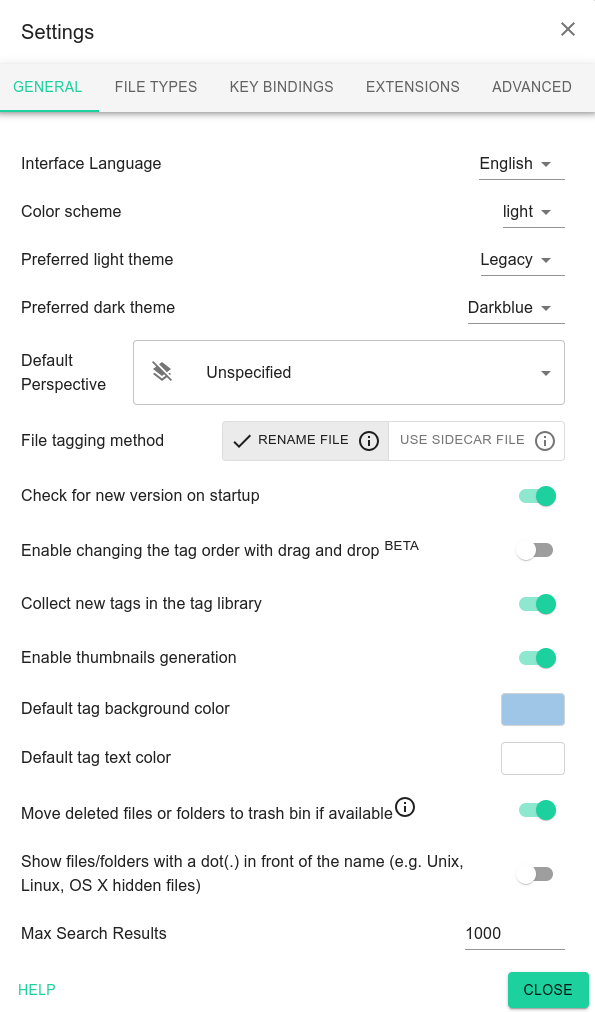The image depicts a settings menu interface with a predominantly white background and black text. At the top of the screen, there are several clickable tabs labeled "General," "File Types," "Key Bindings," "Extensions," and "Advanced." 

Directly beneath these tabs, the interface displays various settings options. The first setting listed is "Interface Language," set to English. Below that, the "Color Scheme" is set to Light. Further down, the "Preferred Light Theme" is specified as "Legacy," while the "Preferred Dark Theme" is "Dark Blue." 

The next section indicates that the "Default Perspective" is currently "Unspecified," with a drop-down arrow suggesting alternative options can be selected. Following this, the "File Tagging Method" is presented, with two choices: "Rename File" and "Use Sidecar File." The "Rename File" option is selected, evidenced by a checkmark.

Additionally, the menu includes various other adjustable settings such as "Default Tag Text Color" and "Enable Thumbnails Generation," each accompanied by sliders. These sliders are color-coded; green signifies that the setting is enabled, while gray indicates it is disabled. 

Finally, a prominent green "Close" button is located at the bottom of the screen, allowing users to exit the settings menu.